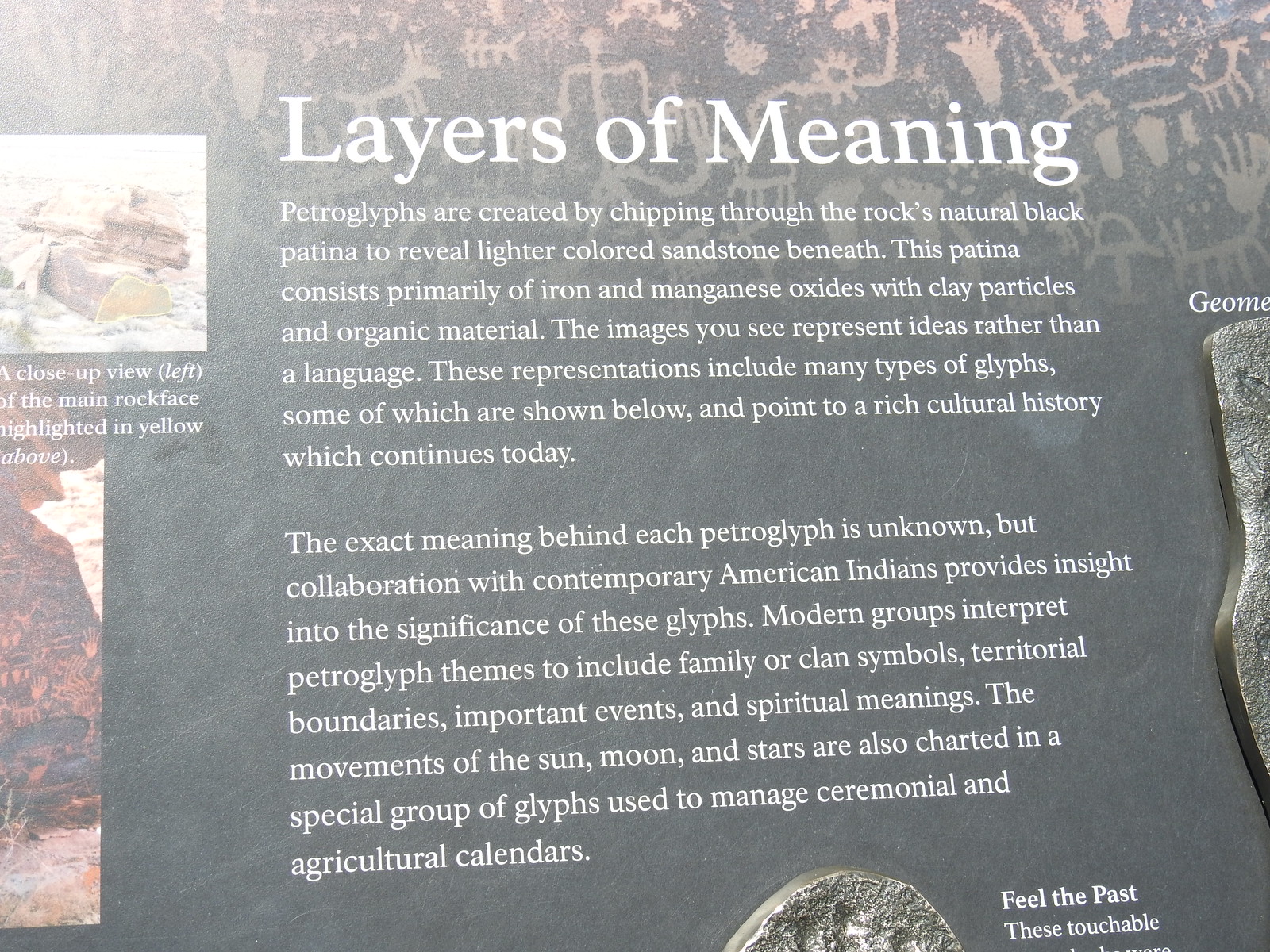The image showcases a gray plaque or poster set against a light, multicolored background, and it occupies most of the frame. The top of the plaque features large white text stating "Layers of Meaning." Below this heading, the text explains that petroglyphs are created by chipping through the rock's natural black patina to reveal the lighter-colored sandstone beneath. This patina, composed primarily of iron and manganese oxides, along with clay particles and organic material, adds to the intricate detailing of the petroglyphs. The inscription delves into the cultural significance of these images, noting that they represent ideas rather than a written language, highlighting their importance in showcasing a rich, ongoing cultural history. 

The plaque mentions how contemporary American Indians help interpret these petroglyphs, providing insights that suggest they symbolize family or clan identifiers, territorial boundaries, important events, and spiritual meanings. Special glyphs also chart the movements of celestial bodies for managing ceremonial and agricultural calendars. To the left of the plaque, there is a small inset featuring a close-up view of a rock face highlighted in yellow. On the right side, partially visible, is a silver shape resembling a bottle, with geometric patterns.